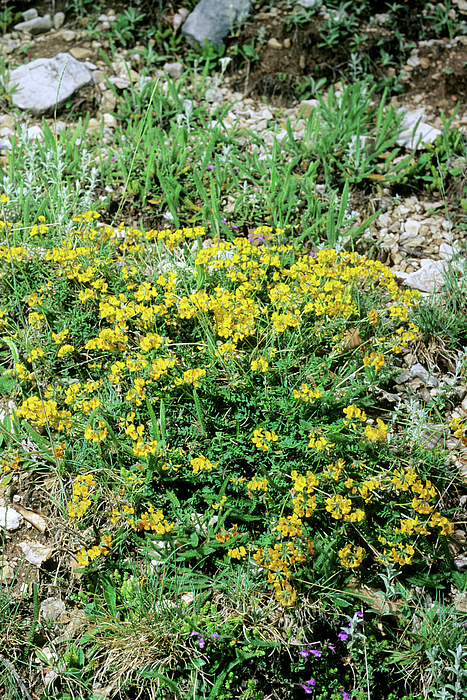The photograph captures a vibrant garden scene in broad daylight, where the focal point is a clump of striking yellow flowers with three to four petals each, clustered together on single stems. Surrounding these yellow blooms are an array of small green leaves and long blades of grass. The image also includes patches of purple flowers that resemble the yellow ones in structure, scattered towards the bottom of the frame. Various bare patches of dark brown dirt and small clumps of pebbles and rocks add texture to the scene, suggesting that water might regularly flow through this area, resembling the bottom of a small creek bed. Notable details include a flat gray rock in the top left and a similar gray rock positioned at the top center. The entire area is bathed in sunlight, showcasing the lush greenery, additional elements like brown twigs, bushes, and white stones, and creating a dynamic natural tableau.